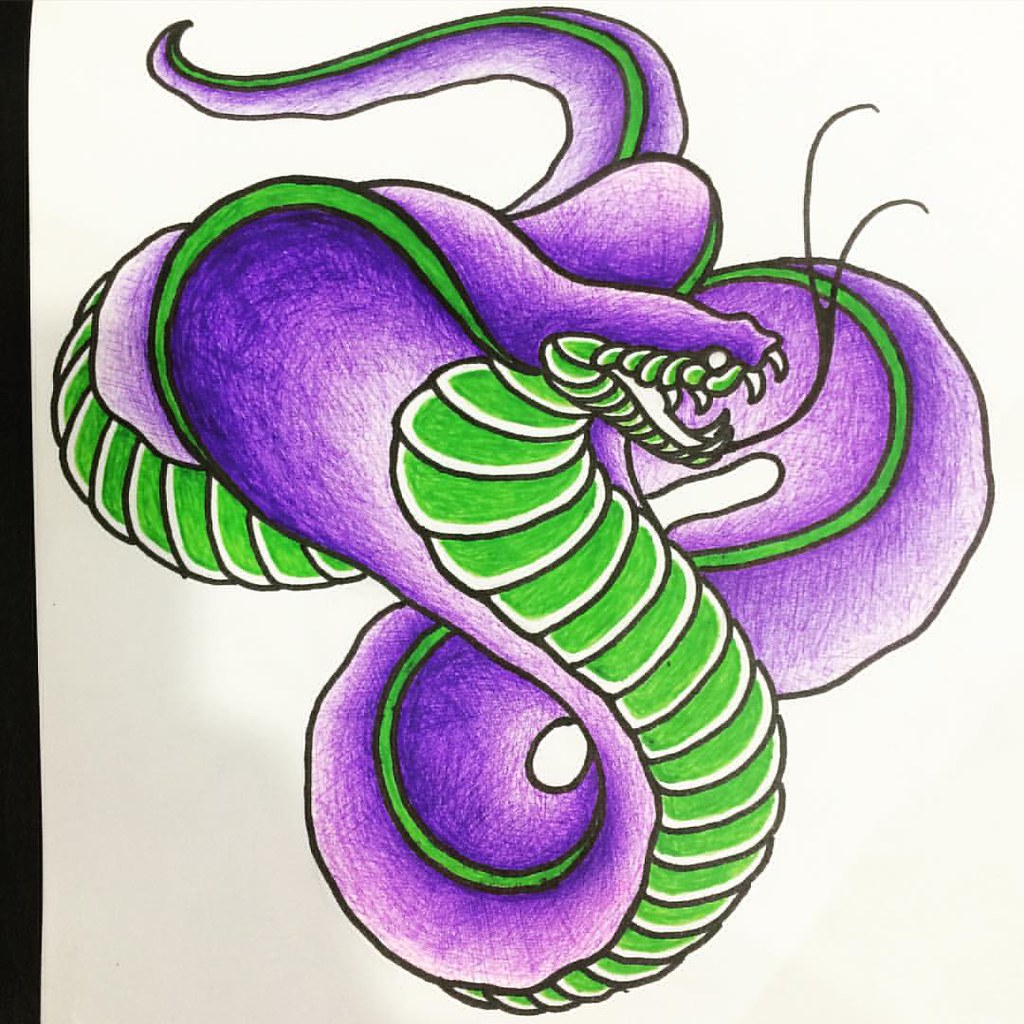This detailed artwork showcases an imposing cobra, depicted with a monstrous flair, coiled several times on a sheet of white paper. A prominent black border runs along the left edge of the paper, framing the scene. The cobra itself is intricately outlined in black ink and filled in with vibrant colored pencil. The fearsome reptile boasts a rich purple hue along its body, accentuated by a thin, vivid green stripe that stretches from its head to the very tip of its tail. The underbelly is meticulously detailed with scaly textures, rendered in a striking kelly green. The cobra's mouth is menacingly open, revealing a sense of aggression, and a long forked tongue, drawn in black, dramatically extends outward before splitting in two. The detailed rendering and vivid coloring bring this fearsome snake to life on the canvas.